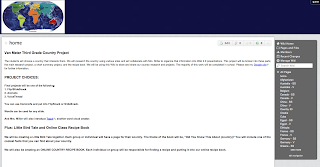This image depicts a website layout. At the top of the page, there is a header featuring a dark blue background adorned with a world map graphic in the upper left corner. Below the header, a large central section with a white background dominates the page, filled with black text that is unfortunately too blurry to decipher. To the right of this central section, there is a tall, vertically-oriented gray box. This box appears to contain categories and other links related to the blog's content. Overall, the website's design appears clean and straightforward, primarily showcasing blog posts.